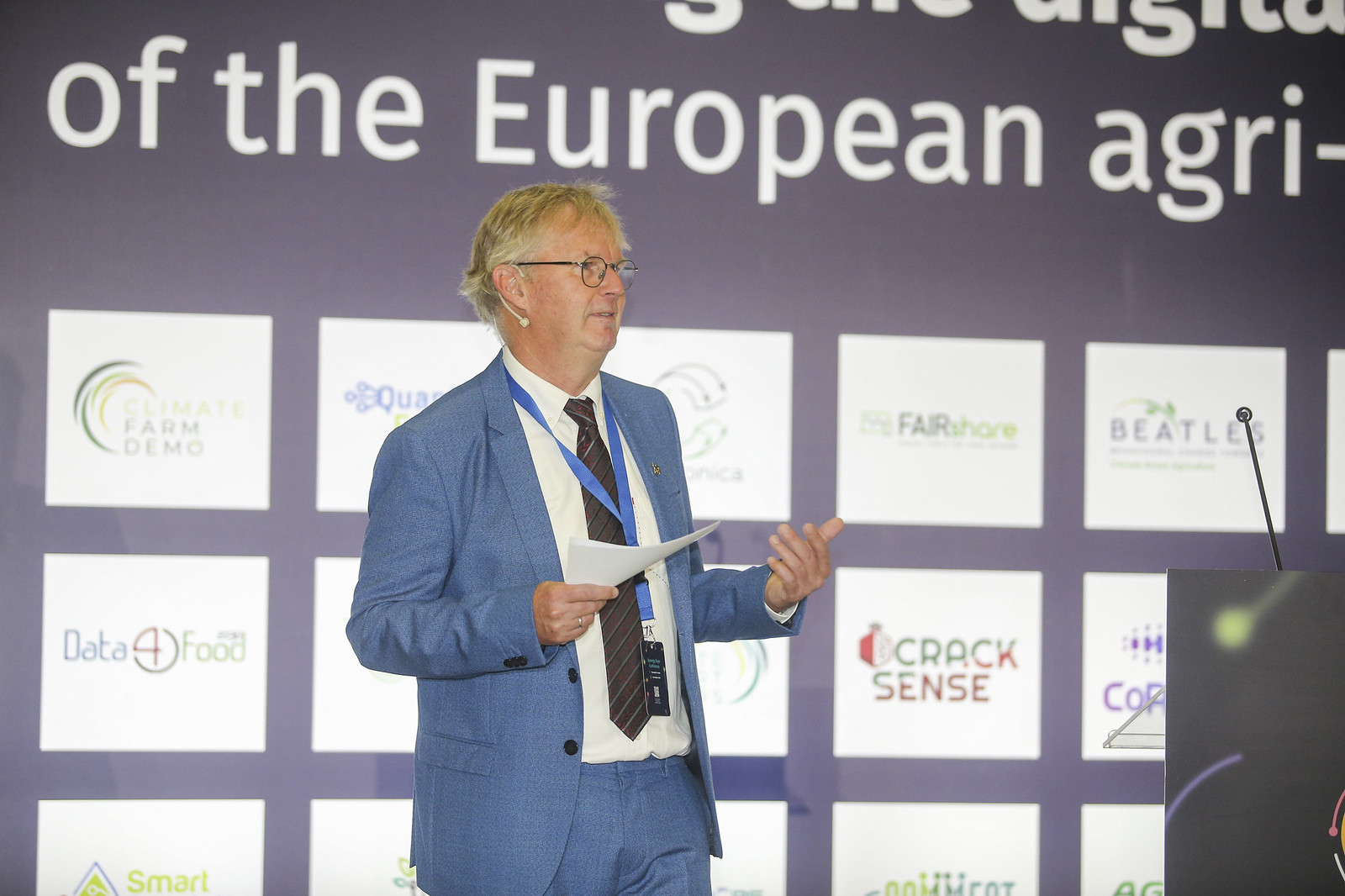In this photo, we see a man, likely in his 50s or 60s, giving a speech or presentation at an event. He has short gray hair, wears glasses, and is dressed in a light blue suit with his jacket open to reveal a white shirt and a gray-striped black tie. He stands in the center of the image, holding some sheets of paper in one hand while the other hand is raised, as if mid-speech.

To the bottom right, a black podium with purple and yellow streaks is visible, with a thin black microphone extending from it, suggesting he is speaking into it. The background features a large screen with the words "of the European Agri-" at the top, though the rest of the text is cut off. Below this, multiple white squares display various company logos, including DataFood, CrackSense, FairShare, Beatles, and Smart something, among others.